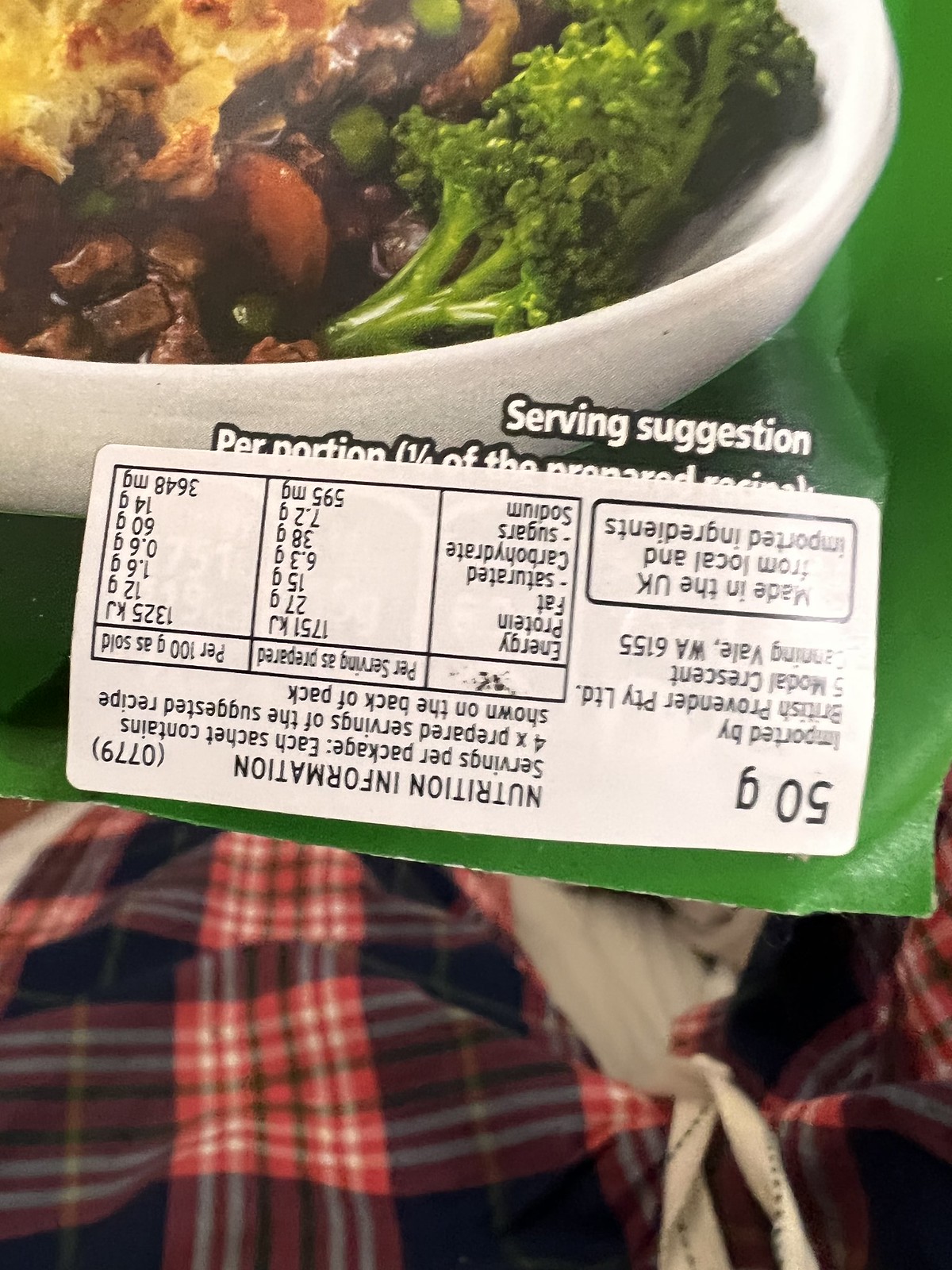A close-up image shows the corner of a food product’s box, primarily focusing on the upper left portion of the packaging. The image prominently features an appetizing depiction of a bowl filled with broccoli, meat, and gravy, which extends from the upper left to the center of the frame. Positioned at the lower right-hand side of the image is an upside-down nutritional label. The legible part of the label indicates "50 grams" on what would be the bottom right side of the image.